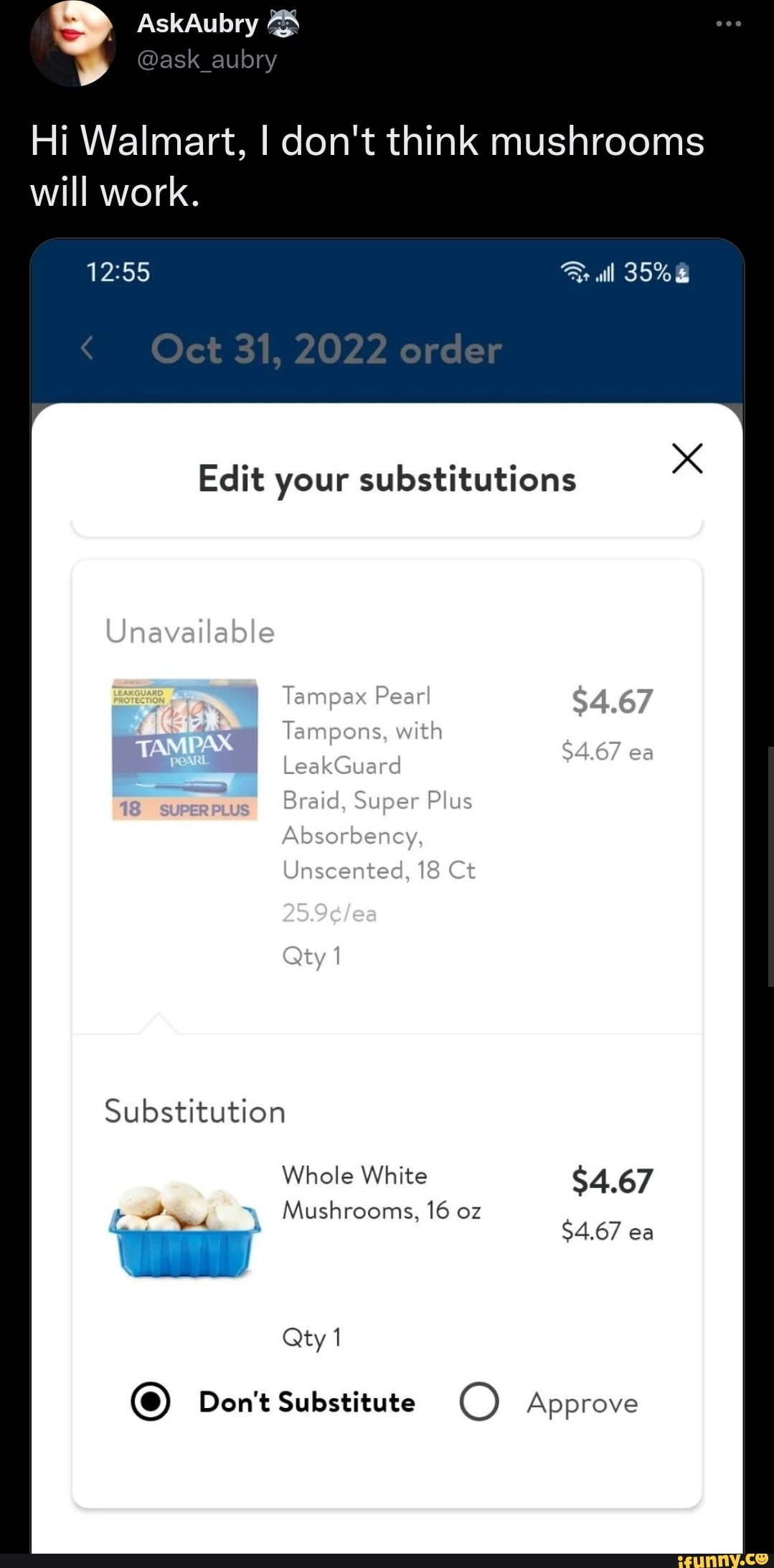This image is a detailed screenshot of a social media post from a mobile device, posted by a user named "@ask_Aubrey." The post humorously addresses Walmart’s item substitution suggestion. The user’s avatar is partially visible, showing the lower half of a white woman’s face with red lipstick, against a black background.

To the right of the avatar, the user’s name "Ask Aubrey" appears alongside a raccoon icon, followed by the handle "@ask_Aubrey." Below, the post text reads, "Hi Walmart, I don't think mushrooms will work."

The screenshot captured within the post depicts a mobile order interface. At the top, a blue bar shows the phone's status, including the time (12:55), Wi-Fi connection, signal strength (showing two bars), battery percentage (35%), and the battery icon. The date displayed is October 31, 2022, alongside the word "Order" and a less-than symbol (<) on the left.

The main content area features an "Edit Your Substitution" pop-up with an 'X' to close it. Listed is the unavailable product: "Tampax Pearl Tampons with LeakGuard Braid, Super Plus Absorbency, Unscented, 18 count," priced at $4.67. The product image is grayed out with the text “Unavailable” above it.

Humorously, the suggested substitution is "Whole White Mushrooms, 16 oz," also priced at $4.67. The image shows mushrooms in a blue plastic container. Below this, there are options to "Don't Substitute" or "Approve," with "Don't Substitute" selected.

This screenshot humorously highlights the mismatch between the original product and the suggested substitution.